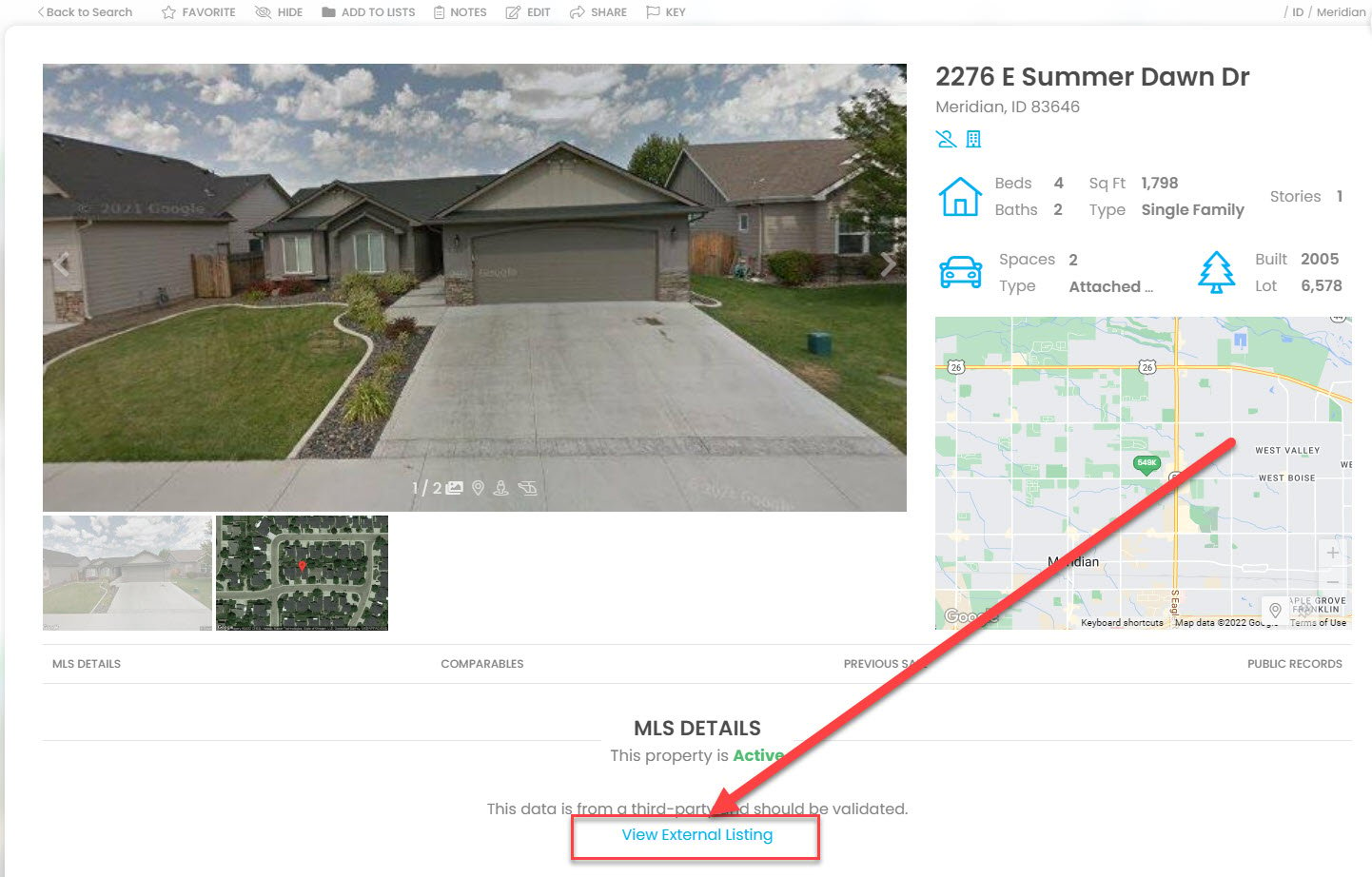A rectangular image features a single-story house with a large driveway and a grass lawn, bordered at the top by a navigation bar that displays options such as "Back to Search," "Favorite," "HOE," "Add to List," "Notes," "Exit," "Share," and "Key." The house has several front-facing windows and is labeled as one of two available images. To the right of the image, text provides detailed information about the property: it is located at 2276 East Summer Dawn Drive, Meridian, ID 83646. The house features four bedrooms, two bathrooms, and has a square footage of 1,798. It is a single-family, one-story home with an attached two-car garage, built in 2005, and situated on a 6,578 square foot lot. Below this information, a map displays the location of the house with a prominent red arrow pointing to the middle, accompanied by a link labeled "View External Listing." The bottom section of the image contains MLS details indicating that the property is active, and notes that the data is sourced from a third party and should be verified.